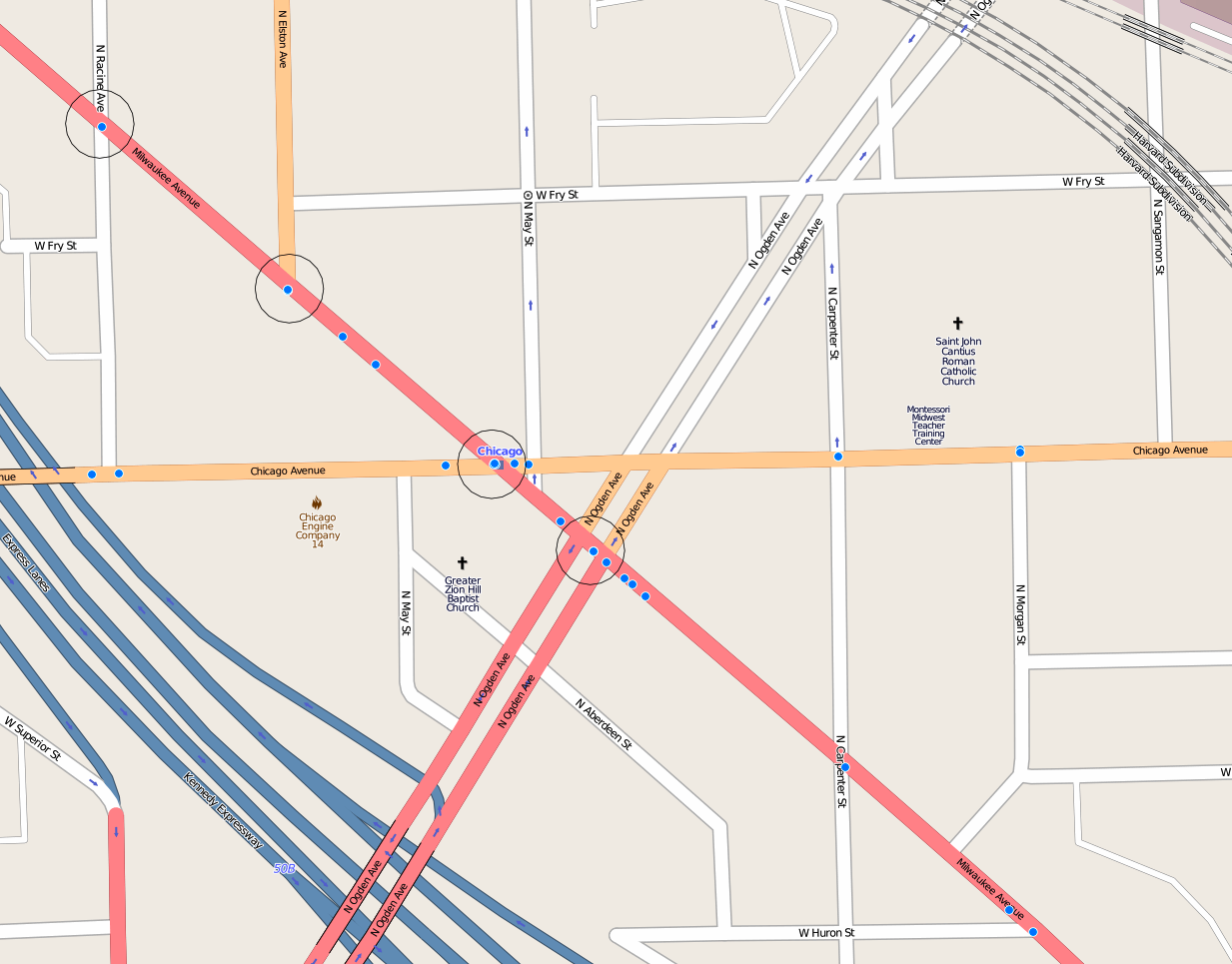This detailed map features what appears to be a section of Chicago, prominently displaying a series of intersecting lines denoting different types of roads and potential transit routes. At the center, running horizontally, is Chicago Avenue, colored in yellow. This major street is intersected by a myriad of other lines, each representing various road types or highways.

A significant diagonal thoroughfare, possibly Milwaukee Avenue, spans from the top left to the bottom right corner of the image and is marked in a distinctive red or pink hue. Along this avenue, several blue dots—many circled—suggest bus stops or similar transit points. These blue dots are also scattered along Chicago Avenue and align with similar stops.

The map includes multiple white streets, adding to the intricate network. Another yellow-hued road, matching Chicago Avenue's color, runs through a section of the map. In the bottom left corner, additional pink lines intersect, suggesting more important routes. Several parallel blue roads originate from the left center and extend diagonally down to the bottom center, interconnecting with other roads.

There are also small dotted lines in the upper right corner whose purpose is unclear due to the lack of a legend or readable labels. This absence of clear identifiers means the exact function of these marks remains uncertain. Overall, the color-coded lines and numerous marked stops give this map a style reminiscent of those found at transit stations, be it for buses or trains, although there are no explicit labels or legends confirming this.